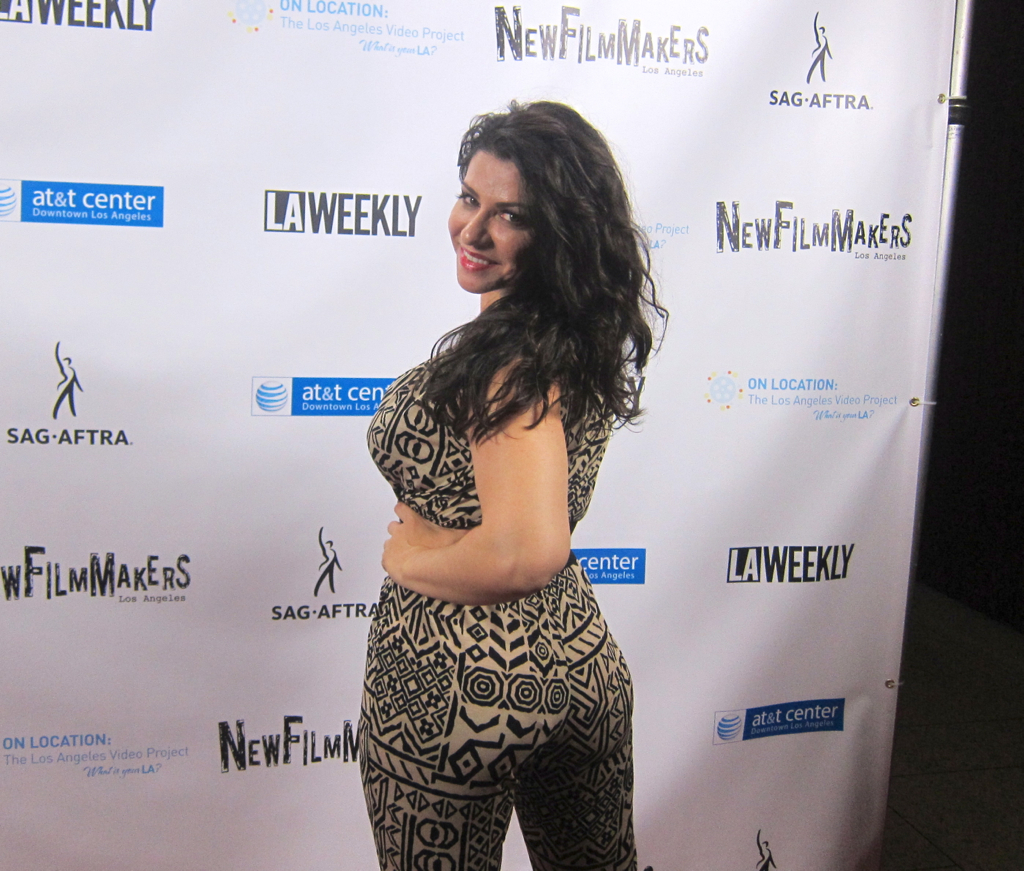In this vibrant indoor photo taken at a Hollywood-type event, an attractive young woman with wavy dark hair cascading past her shoulders stands confidently with her back partially turned toward the camera. She exudes elegance in a short-sleeve, one-piece jumpsuit with a distinctive geometric pattern in black and tan, accentuating her figure. Her radiant smile is highlighted by striking red lipstick, captured as she glances back over her shoulder. The backdrop behind her is a white banner adorned with various logos, including AT&T Center, LA Weekly, SAG-AFTRA, and New Filmmakers, emphasizing the event's significance. To the right, glimpses of the room's interior, including a supporting pole for the banner and sections of the floor and wall, can be seen, adding context to the setting.